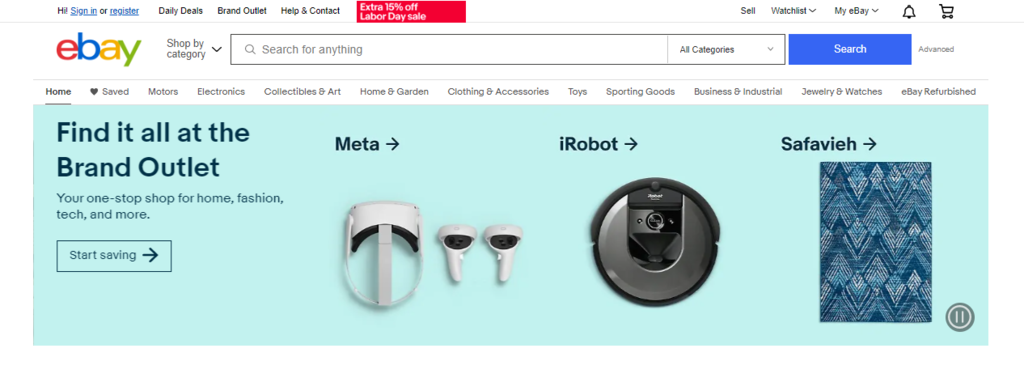The image showcases the eBay website interface. Starting from the top left corner, it greets the user with "Hi," followed by the "Sign in" and "Register" buttons. Next to these buttons are navigation links including "Daily Deals," "Brand Outlet," and "Help & Contact." A prominent green and red banner announces an "Extra 15% off Labor Day" offer. 

At the top right of the page, various user options are visible such as "Set Watchlist," "My eBay," a notification bell, and a shopping cart icon. Just below "Sign in" is the eBay logo. Beneath the logo, there is a "Shop by Category" dropdown alongside a search bar, with an "All Categories" dropdown to its right and a blue "Search" button.
 
Further down, a horizontal menu showcases various categories including "Home," "Saved," "Motors," "Electronics," "Collectibles & Art," "Home & Garden," "Clothing & Accessories," "Toys," "Sporting Goods," "Business & Industrial," "Jewelry & Watches," and "eBay Refurbished."

At the bottom of the screen, a light blue banner features the text "Find it all at Brand Outlet." To the right of this text, there are icons for "Meta," "iRobot," and "Sebaya," each accompanied by a right-pointing arrow. Below the "Meta" text, there are earbuds depicted; below "iRobot," a small vacuum cleaner is shown; and under "Sebaya," there appears to be a blue carpet with a diamond pattern.